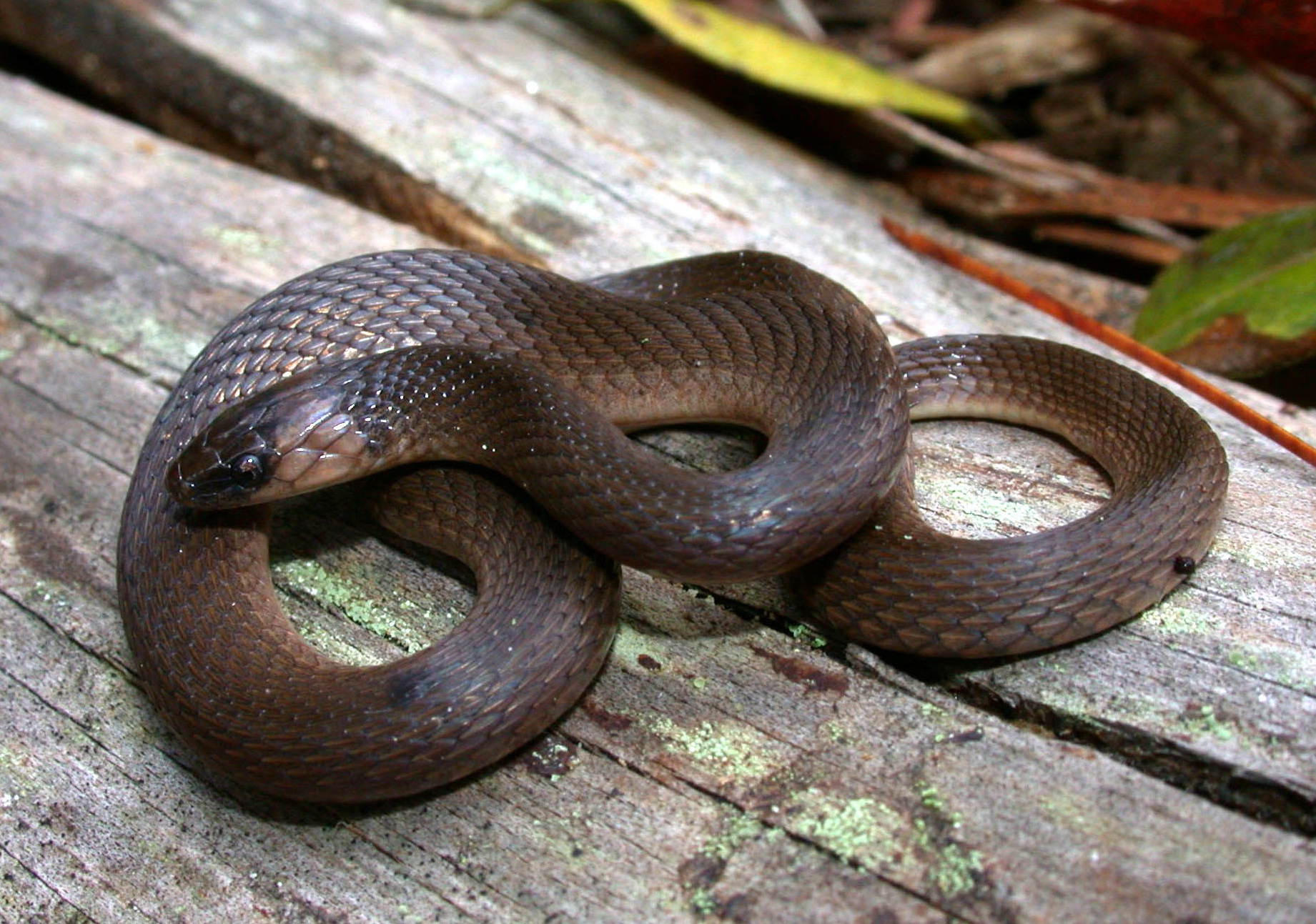In this detailed, horizontally-oriented photograph, a small brown snake, around 3-4 feet in length, is the central focus as it rests coiled up on a piece of aged, moss-covered wood. The snake’s textured, scaly skin and single visible dark eye stand out prominently against the log it sits upon. The snake forms a figure-eight shape with its body, with its head emerging from the coils and facing west. The weathered wood, possibly part of a fallen tree or aged debris, exhibits green patches of moss and is split at both ends, adding to the rustic environment. In the background, blurred elements such as dead leaves and branches hint at a forest floor setting, creating a natural, tranquil scene where the snake remains still, seemingly at ease on its mossy perch.